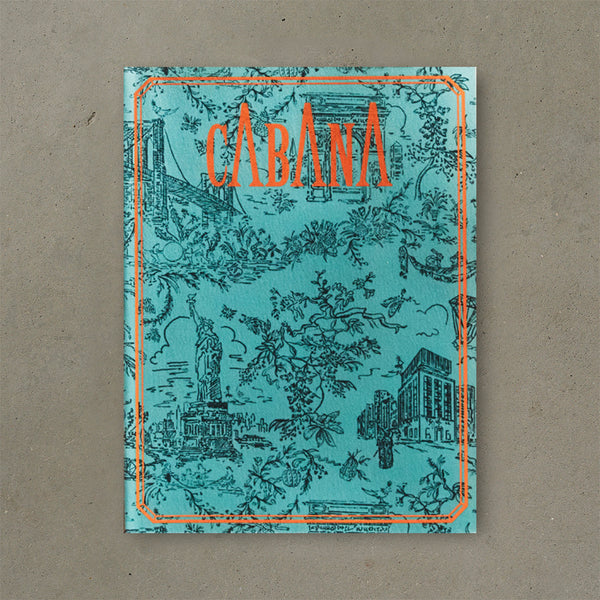The photograph features the cover of a magazine titled "Cabana" with a teal-blue background positioned on a dark gray, cement-like surface. The word "Cabana," prominently displayed at the top center in bold orange serif font, features unusually tall A's resembling upside-down V's. The cover is bordered by a bright, almost neon orange outline. Illustrations in black adorn the cover, including landmarks such as the Brooklyn Bridge, Statue of Liberty, Arc de Triomphe, and, possibly, the Golden Gate Bridge. Decorative floral elements, as well as images of leaves, clouds, an apple, and a bird, enrich the intricate design. The overall composition blends architectural and natural motifs, creating an engaging and visually striking magazine cover.